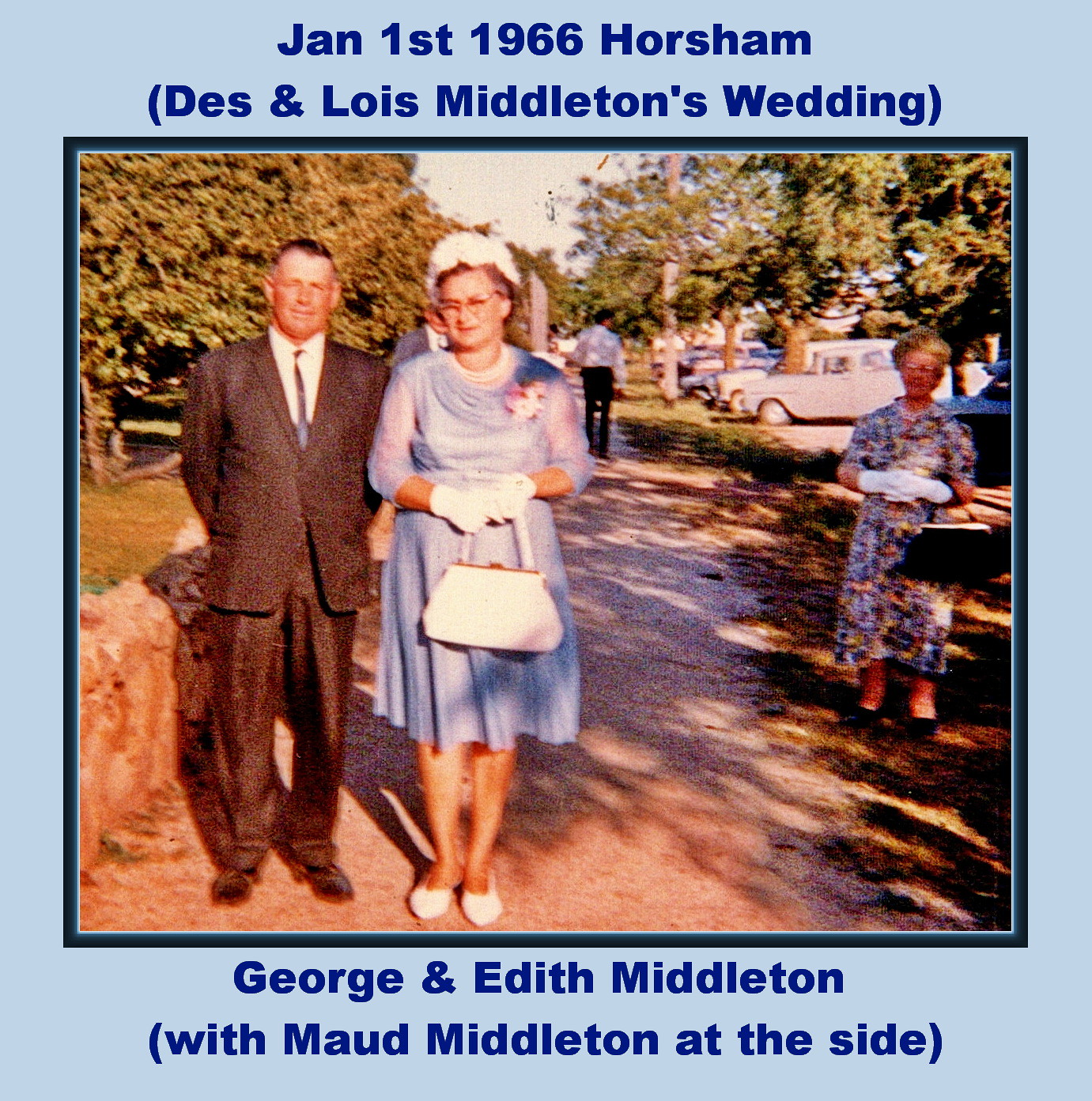The framed photo, bordered in light blue, is a vintage image taken on January 1st, 1966, in Horseham, capturing a moment from Des and Louise Middleton's wedding. The text on the photo reads, "January 1st, 1966, Horseham" and "Des and Louise Middleton's wedding" at the top, and "George and Edith Middleton, with Maude Middleton at the side" at the bottom. The man on the left, likely George Middleton, is dressed in a suit with a skinny tie, and he appears well-groomed, his hands poised behind his back. Standing beside him is Edith Middleton, who is dressed in a proper blue dress, adorned with white gloves and a white bonnet, completing her attire with white shoes and a white purse held in her hands. To the far right stands Maude Middleton, an elderly woman, likely around 60 to 70 years old, wearing a colorful floral dress, with white gloves and a black purse on her wrist. The backdrop features several people, old cars parked in the background, and surrounding trees, complementing the timeless quality of the slightly aged photograph.